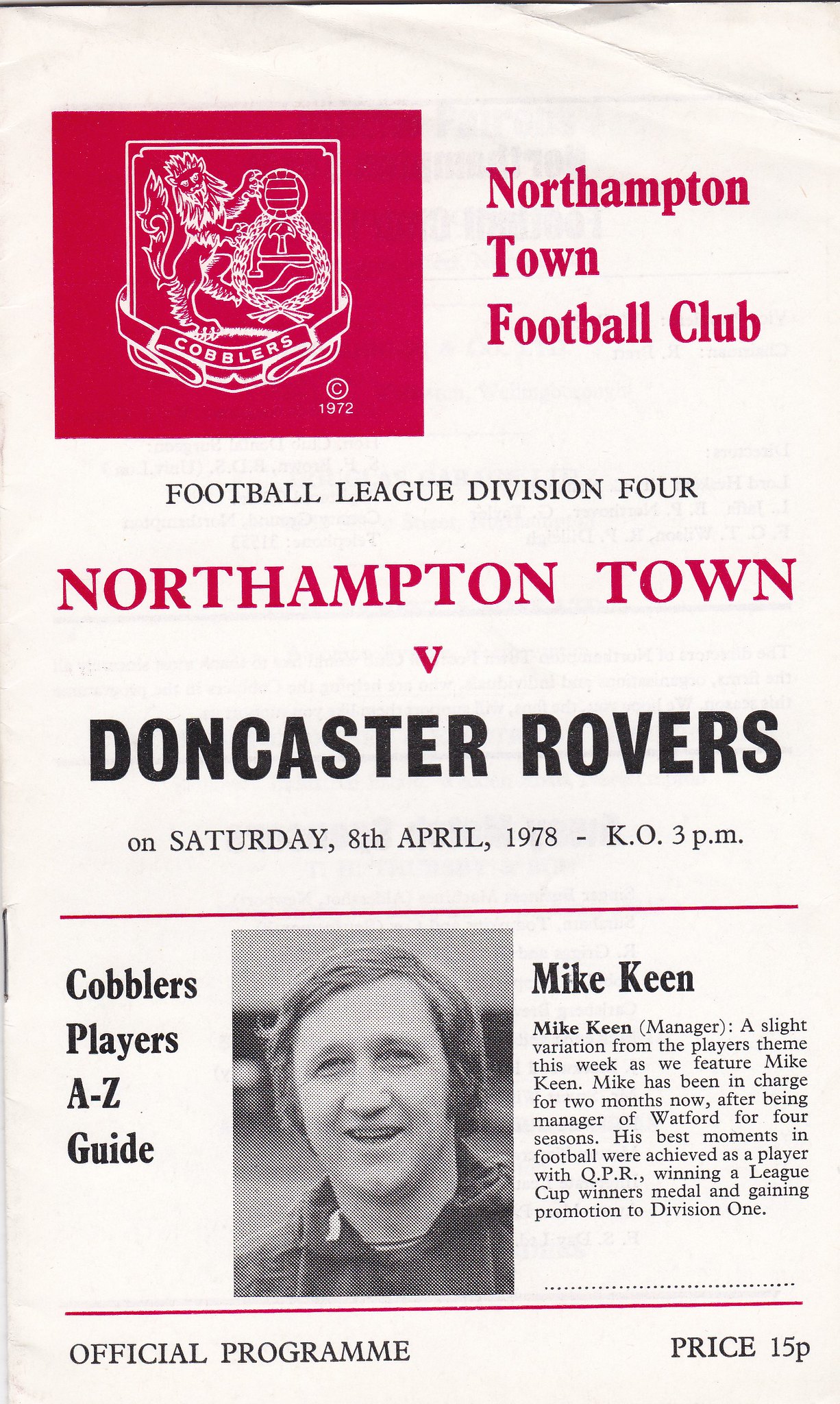The image depicts an old program from Northampton Town Football Club, featuring text in black and red on a white background. At the top, there is a red square with an emblem in the center, showcasing a lion within a shield and the word "Cobblers" beneath it. To the right of this emblem, the header displays "Northampton Town Football Club" in red letters. Below this, "Football League Division 4" is printed in black, and beneath it, in red, "Northampton Town V Doncaster Rovers" is noted. The details include the date "Saturday, 8th April 1978," with a kickoff time at "3 p.m."

Further down the program, separated by a red line, there is a section titled "Cobblers Players A to Z Guide." Adjacent to this title is a black-and-white photograph of a man, identified as Mike Keene. To the right of the photograph, a description states that Mike Keene is the manager. The synopsis elaborates that Mike has been managing for two months, following a four-season tenure as Watford’s manager, and highlights his successful football career as a player with QPR, where he won a League Cup and achieved promotion to Division One. At the bottom, another red line precedes the text "Official Program, Price 15p."